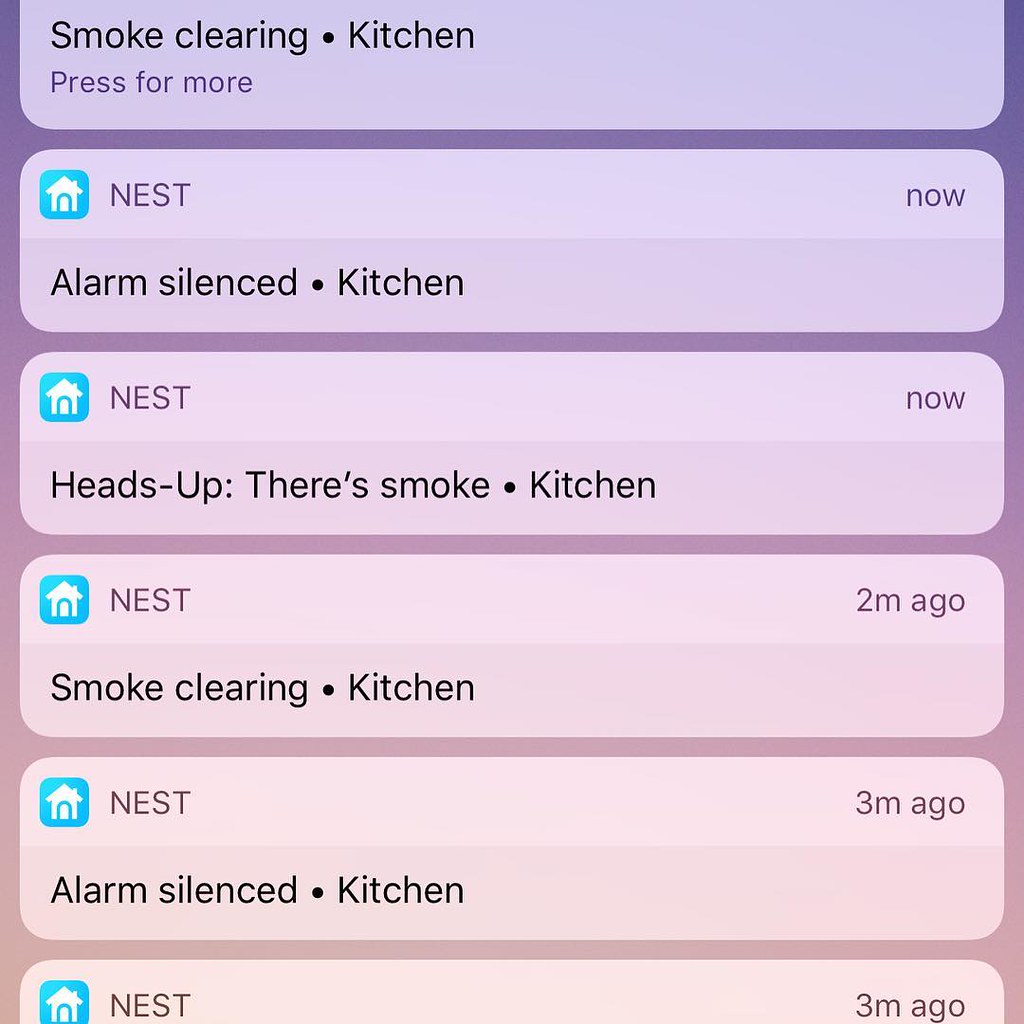A detailed close-up screenshot taken from a smartphone displaying a series of notifications from a Nest smart thermostat. The notifications appear to be related to an incident in the kitchen, likely triggered by cooking activities. The sequence starts with a notification from three minutes ago stating, "Alarm silenced - Kitchen," followed by a two-minute-old notification indicating, "Smoke clearing - Kitchen." More recent notifications then appear, including two brand new alerts that read, "Heads up, there’s smoke - Kitchen," and another immediately stating, "Alarm silenced - Kitchen." The sequence concludes with another message saying, "Smoke clearing - Kitchen." The older notifications at the bottom are partially cut off, making them unreadable. The series of alerts suggests that the Nest smart thermostat has been actively monitoring and reacting to smoke detected in the kitchen area.